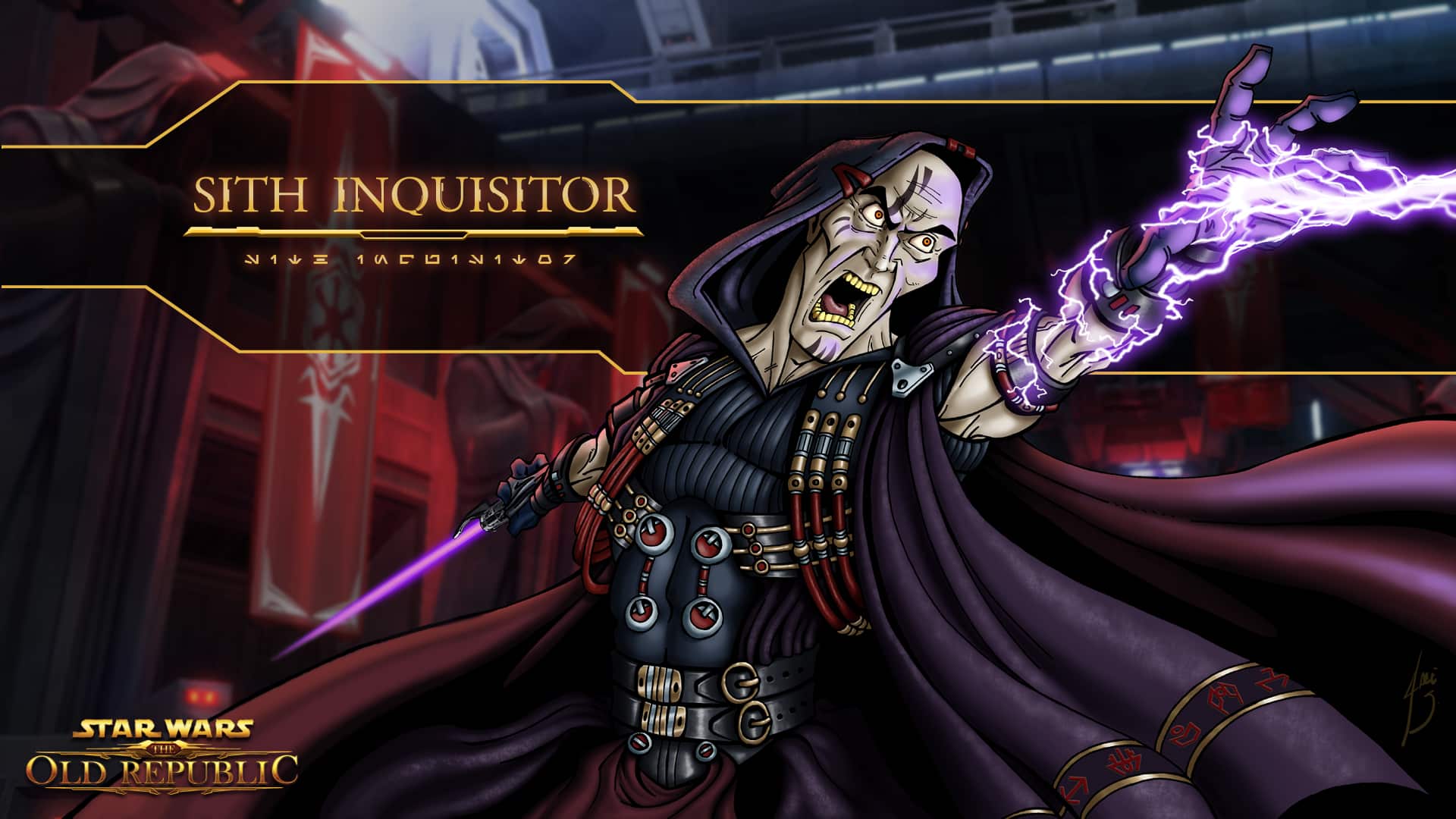This is an ad for Star Wars: The Old Republic featuring an animated, artist-rendered image of a Sith Inquisitor. The character is depicted with gray skin and a hooded, dramatic black cloak billowing as if caught in the wind, worn over a black muscle suit adorned with red straps, buckles, and metallic attachments, giving it a steampunk aesthetic. The cloak has deep maroon or purple hues with insignias and gold stripes at the bottom. The Sith Inquisitor, pushed to the right side of the image, wields a purple lightsaber in his right hand, while his left hand is extended outward and upward, emitting purple electrical energy that crackles from his glove. Behind him, a banner reads "Sith Inquisitor," and to the bottom left, the ad is labeled "Star Wars: The Old Republic." The background sets the scene inside a red-lit facility resembling a warehouse or factory, complete with large structures and a blue-colored walkway.